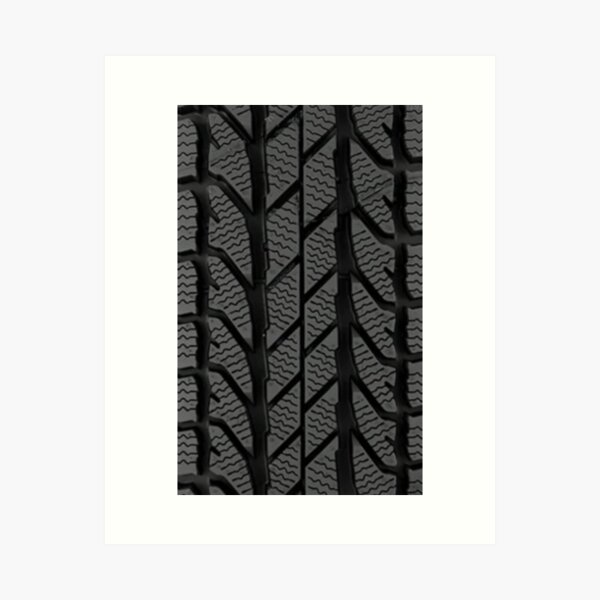The image depicts a highly detailed, zoomed-in close-up of brand new tire tread within a rectangular box framed in white. The tread features a modern, intricate design with four vertical lines from which smaller diagonal lines emanate outward, forming geometric boxes. Inside each box are squiggly lines, enhancing the textured appearance. The tire’s grooves and sections are meticulously etched, maintaining consistent width and depth throughout despite their varied sizes. The overall color scheme is gray and black, showing the clean, unmarred rubber surface typical of tires fresh from the lot.